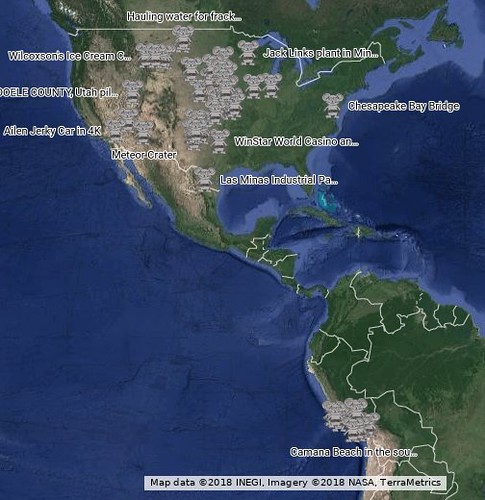The image is a detailed digital satellite map resembling those from Google Maps, covering the United States, parts of Canada, and extending into South America. The map features blue oceans and a mix of green and brown terrain for the continents. Each country is outlined in white, with the title "Hauling Water for Frack..." at the top. Superimposed on the map are various text labels including "Wilcoxon's Ice Cream," "Chesapeake Bay Bridge," "Jack Link's Plant in MIN," "Winstar World Casino," "Laminas Industrial P.A.," "Comana Beach in the south," "Meteor Crater," "Dole County, Utah," "P-I-L," and "Alien Jerky Car in 4K." Notably, gray cartoon koala-like critters are scattered across the map, mainly in the central U.S. and the west side of South America, without a direct one-to-one correlation with the textual labels. At the bottom, there is a white bar with black text reading "Map data 2018 INEGI Imagery 2018 NASA TerraMetrix."